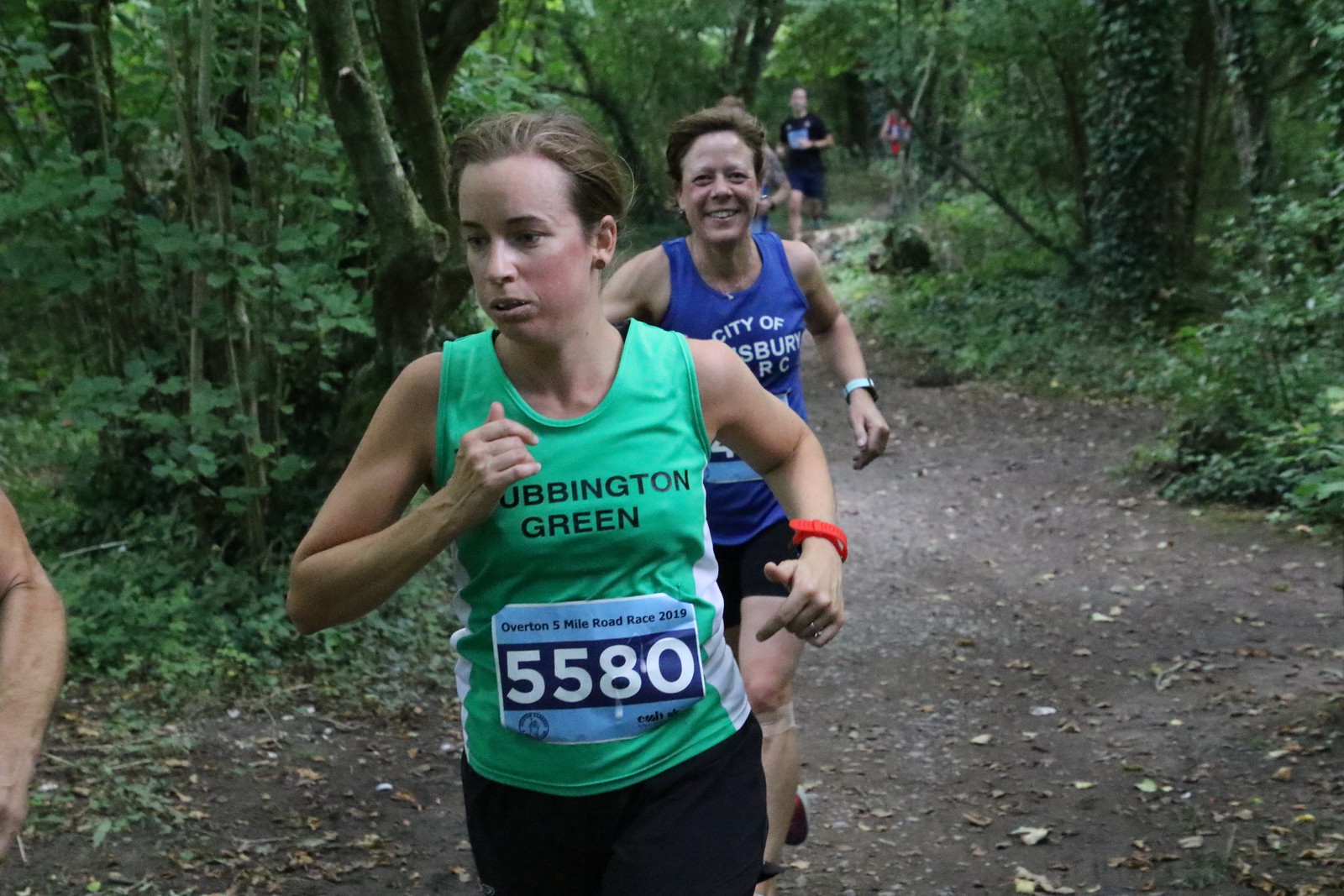The image depicts a group of runners participating in the "Dubbington Green Overton five-mile road race 2019" as they traverse a lush, wooded trail. The focal point is a white woman in the foreground with brunette hair, wearing a sleeveless green shirt bearing the race details and number 5580. She sports a red watch or tracking device and black running shorts, captured in a strong running stride. Directly behind her is another white woman of similar build, donned in a blue tank top with a different city name and black shorts, her blonde hair tied back neatly. In the background, additional runners, including both women and men, can be seen making their way along the dark brown dirt path surrounded by dense greenery, trees with climbing vines, and vibrant leaves.